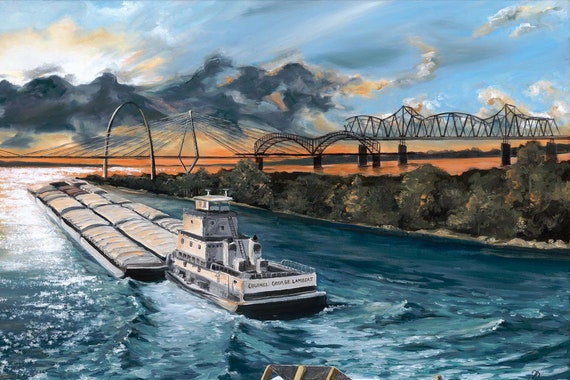This vividly lifelike oil painting captures a dynamic river scene, possibly reminiscent of industrial riverways like those in Pittsburgh, though its precise location is uncertain. Dominating the composition is a powerful tugboat pushing a barge laden with cargo concealed under white tarps. The waterway, clear and blue, may be a canal or river, bordered by vegetation-rich jetties that add a natural frame to the industrial activity. 

A striking suspension bridge with sharp, triangular lines shares the background with two other distinct steel bridges, juxtaposing modern engineering against nature. Adding to the complexity, a structure resembling the St. Louis Gateway Arch rises near the shoreline. The sky above is a picturesque blend of dark storm clouds and brilliant hues of sunset or sunrise, with deep blues at the zenith and warm oranges and reds illuminating the horizon. This scene, rich with contrasts and details, offers a powerful glimpse into the intersection of nature and human endeavor.